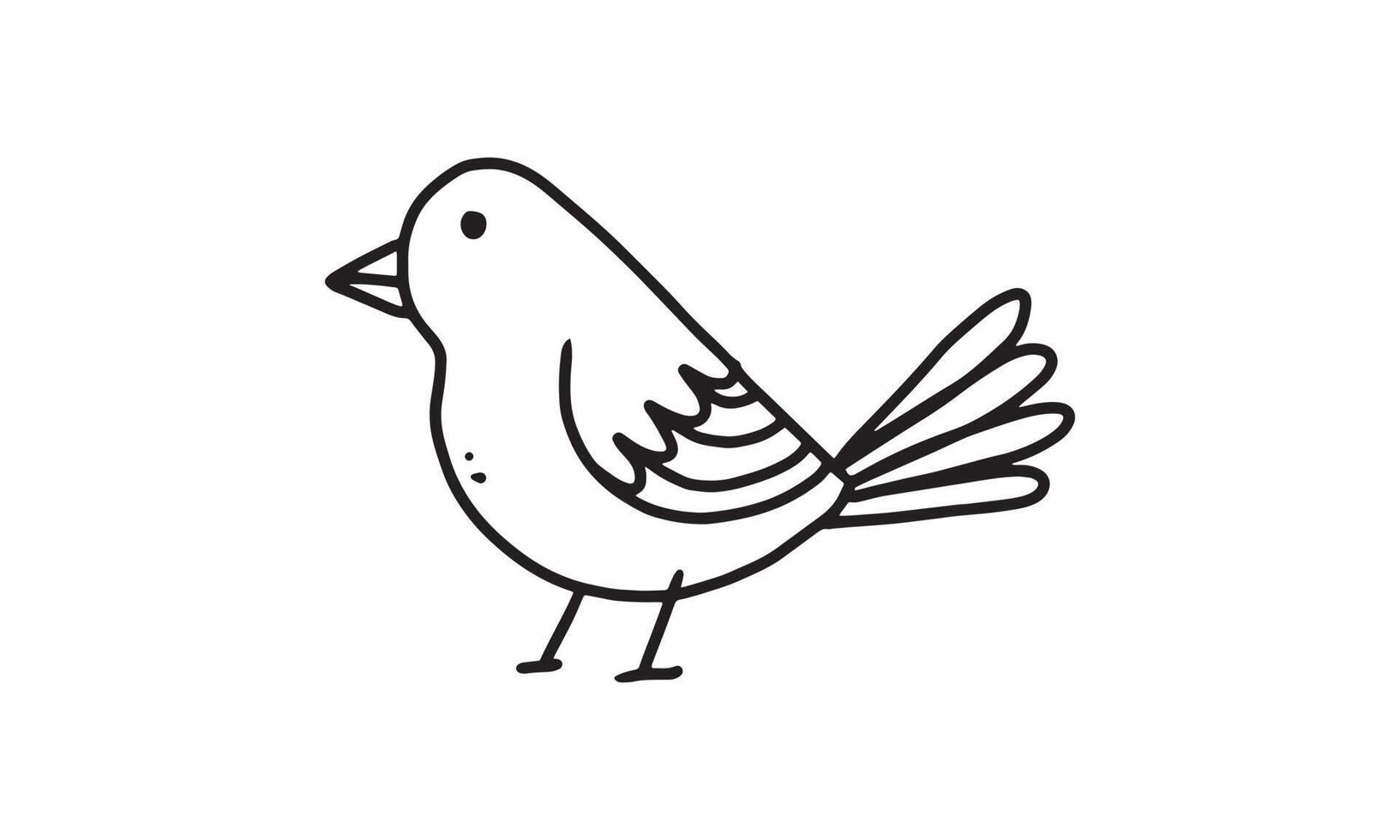This image showcases a hand-drawn, black-and-white cartoon bird against a clear white background. The bird, depicted in a simple ink line drawing, faces left with a pointed triangular beak. Its design consists of a rounded head seamlessly connected to a rounded body. The bird's side view prominently displays a small dot for an eye and two additional smaller dots on its chest, adding depth and character. Its back features a straightforward line, with a wing sketched in an arch adorned with looped-like feathers. The tail extends with four elongated feathers resembling arrows or sausages. The bird's legs are minimalistic, represented by two stick-like lines ending in single horizontal dashes to suggest feet. This plain but charming illustration could easily serve as an icon or logo, encapsulating the essence of a simple, unembellished bird in flight.